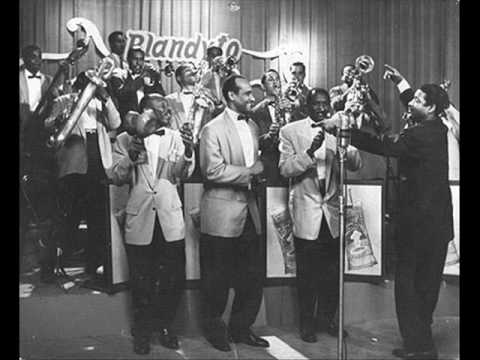The black-and-white photograph depicts a vibrant scene of an African-American orchestra featuring approximately 10 to 12 musicians arrayed across the image. Central to the composition is a conductor positioned on the right side, donned in an all-black suit—jacket and trousers—energetically directing the ensemble with expressive hand movements. The musicians are distinguished by their attire: light-gray jackets with white shirts and black bow ties, paired with black trousers and shoes. 

In the forefront, three individuals seem to be singers, standing out against the backdrop. Behind them, the orchestra’s musicians are engaged with a mix of big band instruments such as trumpets and flutes. Noteworthy is the clear spatial divide between the singers and the instrumentalists, adding depth to the scene.

Framing the image are thin black bands running along the left and right edges, lending a vintage aesthetic. The room is dressed with a dark gray curtain interspersed with white accents, and faint lettering in the upper left corner hints at the word “Blandito” or “Plandito,” adding a touch of mystery to the setting. This collective portrayal suggests a formal performance, perhaps part of a show, characterized by the poised and dynamic stance of the conductor and the meticulous arrangement of the musicians.